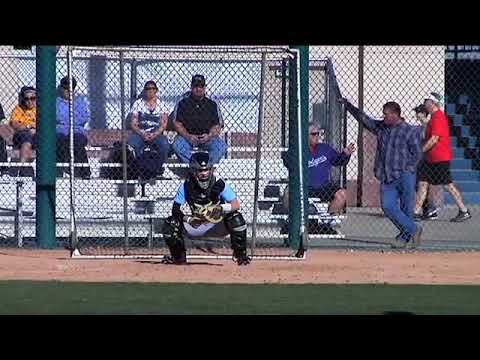The image captures a daytime baseball game scene, rich with details and activities. In the foreground, a catcher in a traditional squatted position, donning a blue shirt, black chest guard, black helmet, knee guards, shin guards, and shoes, is poised behind a netted fence. The catcher, with a mitt ready, is surrounded by parts of the green fence with thick black borders at the top and bottom. Behind the net, a mix of spectators is visible: some are seated on bleachers, while others stand around or walk by. Particularly notable is a man in a plaid blue and gray shirt, leaning casually against the fence with his right arm extended, legs crossed, and engaged in conversation with a person in a long-sleeved blue shirt and black shorts on the bleachers. Additionally, a figure in a red shirt, black shorts, and shoes is walking towards the left side of the image. The scene is brightly lit with natural daylight, emphasizing the vibrant colors and dynamic interactions.